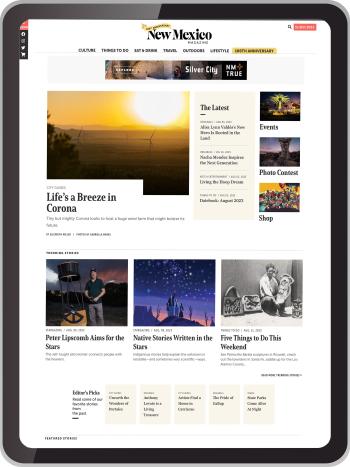This screenshot appears to be taken from a tablet-sized device encased in a black and gray exterior. The image captures a webpage with a white background featuring "New Mexico" prominently at the upper center. Below the header, a navigation menu is visible, though the details are too small to decipher. Directly beneath the menu is an advertising banner for Silver City.

On the left side of the page, there's a vibrant image of a sunset with wind turbines silhouetted in the background. The accompanying caption reads, "Life's a Breeze in Corona." Adjacent to this image on the right, a section titled "The Latest" displays several headlines.

Further to the right, three images with captions are arranged vertically under distinct categories: "Events," "Photo Contest," and "Shop." Positioned below this section, three photos are aligned side-by-side. Their respective captions read: "Peter Lipscomb Aims for the Stars," "Native Stories Written in the Stars," and "Five Things to Do This Weekend."

At the very bottom of the screen, there is a segment labeled "Editor's Picks," featuring five yellow squares arranged horizontally, each containing text.